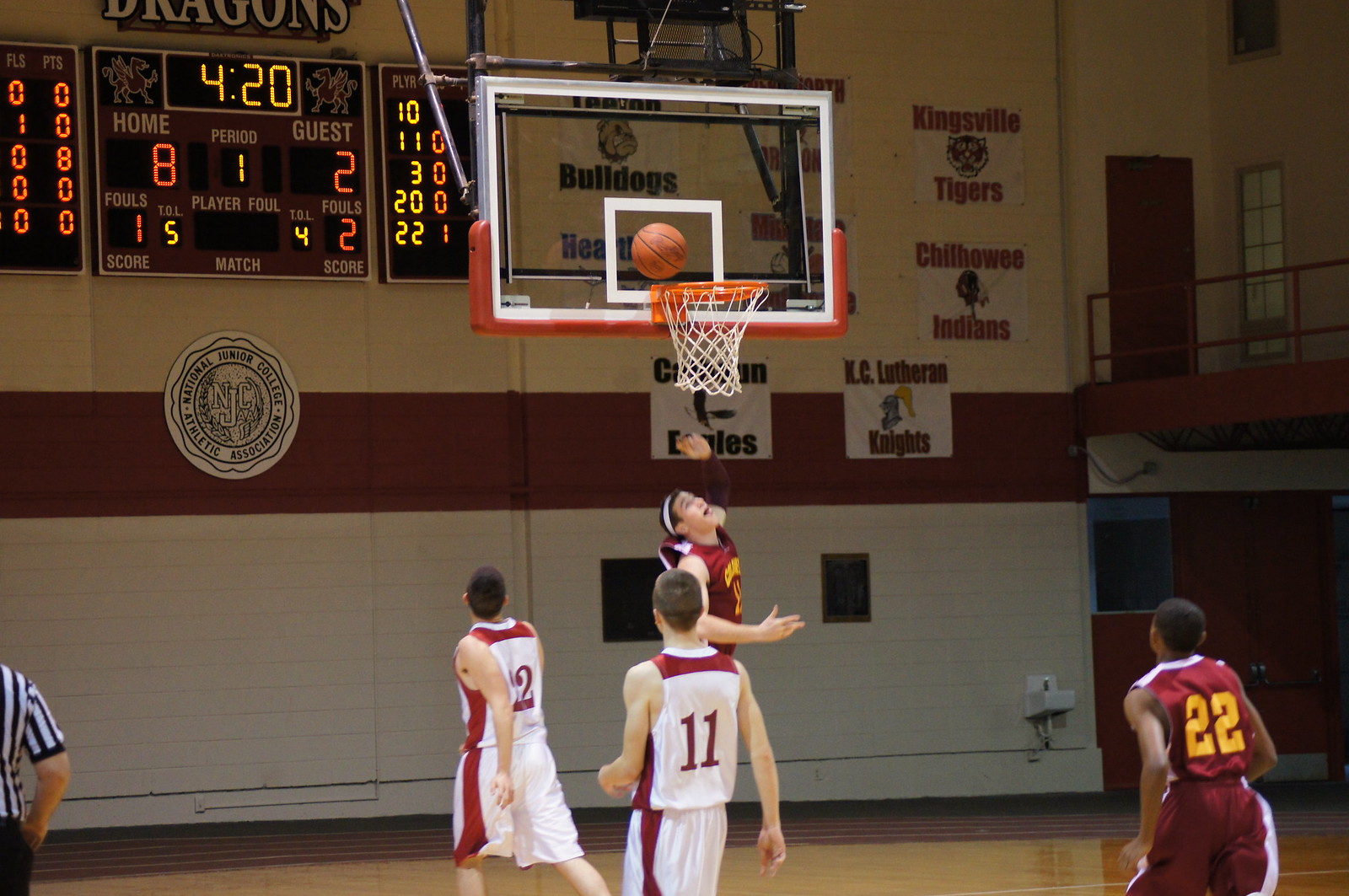In this high school indoor basketball game, the action unfolds on a gymnasium court between two teams: one clad in burgundy with white accents, and the other in predominantly white with burgundy details. The burgundy team's jerseys feature yellow text, while the white team's jerseys have red text for the numbers. A player from the burgundy team is mid-layup, with the ball poised just off the backboard. The scoreboard in the background shows 4 minutes and 20 seconds remaining in the first quarter, with the home team leading 8-2. Additionally, the scoreboard notes one foul for the home team and two for the guests. The gym is detailed with white walls and red stripes, a second-floor balcony on the right, and a water fountain at the bottom right. A referee in a traditional striped uniform stands near the edge of the court. The school hosting the game appears to be Kingsville Tigers, indicated by signs next to the scoreboard.